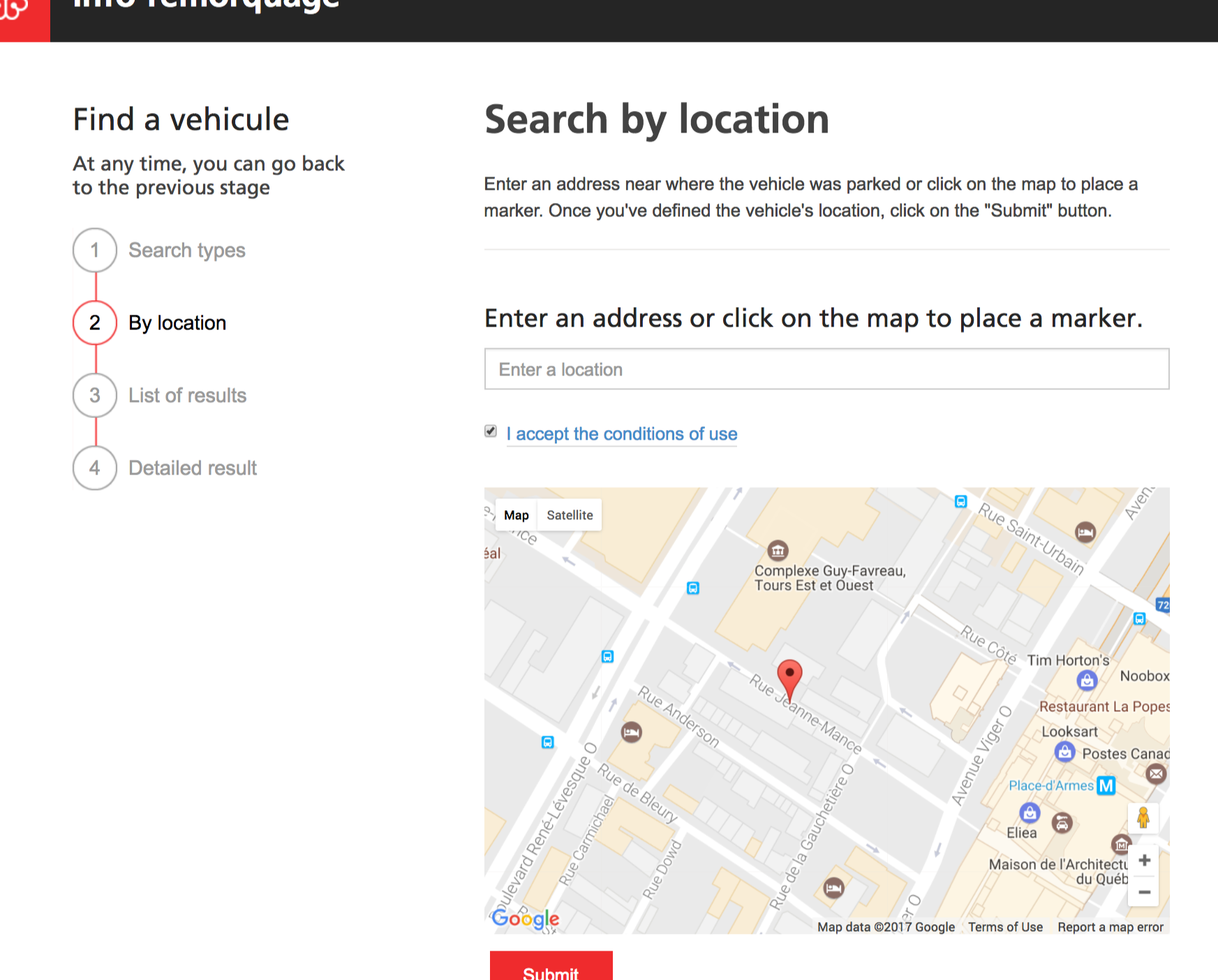The image displays a website interface. At the top left corner, there is a red square with an indistinct white symbol inside it. The top of the screen features a black bar with some white text that appears to say something like "homepage." The detailed visual hierarchy of the interface begins below this bar.

On the left side, there is a navigation option titled "Find a Vehicle," rendered in black text. Below this is a step-by-step progress tracker:
1. **Search by Types** - This is marked by a gray circle with the number "1" and is connected by a red line to the next step.
2. **Location** - This step is currently active, indicated by a red circle with a black number "2."
3. **List of Results** - Represented by a gray circle with the number "3" and is connected via a red line to the next circle.
4. **Detailed Result** - Signified by a gray circle with the number "4."

On the right side of the screen, the active section "Search by Location" prompts the user to enter an address near where the vehicle was parked or to place a marker on a provided map. Instructions detail that after defining the vehicle's location, clicking the "Submit" button is necessary. There is an input box for typing an address and a checkbox with the text "I accept the conditions of use." Below these elements, an image of a Google Map interface is displayed, and at the bottom, a red tab contains the word "Submit" in white text.